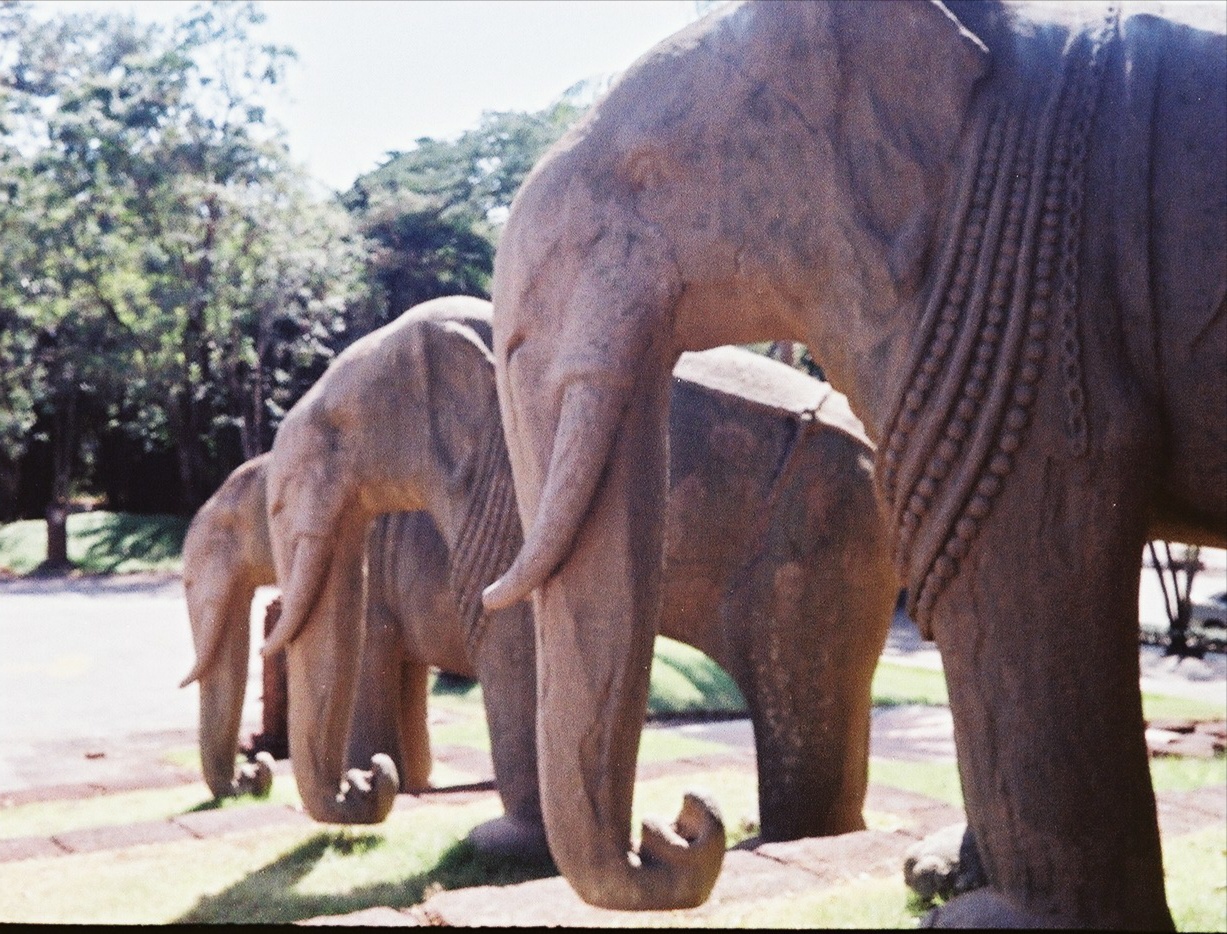The photograph, likely an older scanned or re-photographed print, depicts an outdoor scene on an overcast day featuring three large, intricately carved elephant statues arranged on staggered steps. The statues, with their reddish-brown coloring accented by patches of grey and black, stand on a series of progressively descending steps made from reddish-brown tiles interspersed with green grass. Each elephant is adorned with decorative beaded necklaces draped around their necks and partially over their front legs. The elephants, facing left with their trunks curled upward in a U shape, have tusks and are positioned in a slight diagonal away from the viewer, giving a sense of depth. The photograph captures a mix of natural and manmade elements with the elephants set against a backdrop that includes distant trees, reinforcing the outdoor setting. A thin black strip along the bottom edge of the image hints at the photograph's physical origins.